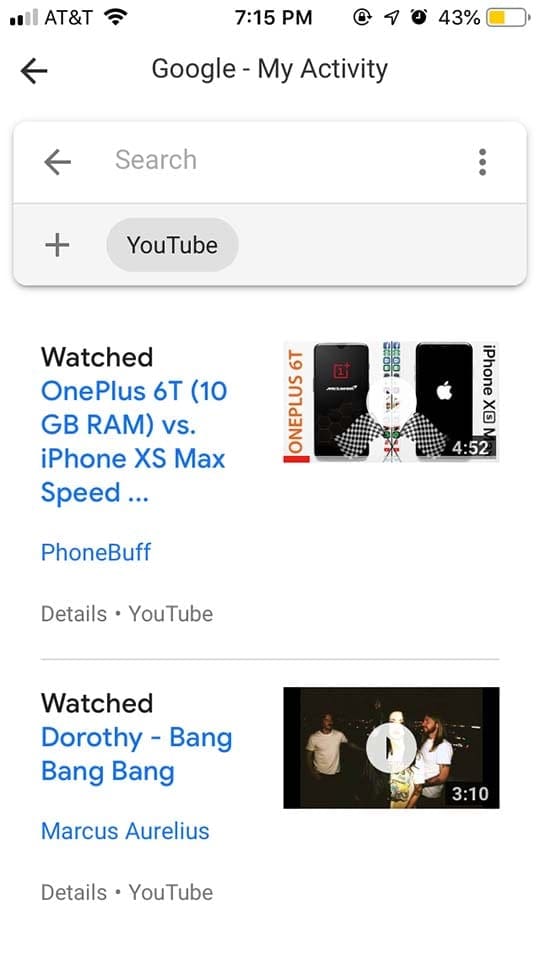This image is a detailed screenshot taken from a mobile device, identifiable by the visible status bar and the rounded shape of a typical cell phone screen. In the upper right corner, the battery indicator shows a 43% charge. Adjacent to it, icons indicate that an alarm is set, location services are active, and it's currently 7:15 PM. The carrier is AT&T, with full WiFi signal strength but only two bars of cellular service.

The main interface depicted is the "Google My Activity" page, presenting a white background with "Google My Activity" written in black text next to a leftward-pointing arrow. Beneath it, a search bar is accompanied by another leftward-pointing arrow and a three-dot hamburger menu. Further down, a plus sign appears next to a grey button labeled "YouTube."

Below these elements, there are thumbnails for two watched YouTube videos. The first video thumbnail is titled "OnePlus 6T 10GB RAM vs. iPhone XS Max Speed" from the channel Phone Buff, and is marked as "watched." The second thumbnail below it is for the video "Dorothy Bang Bang Bang" uploaded by Marcus Aurelius Uploader, also marked as "watched."